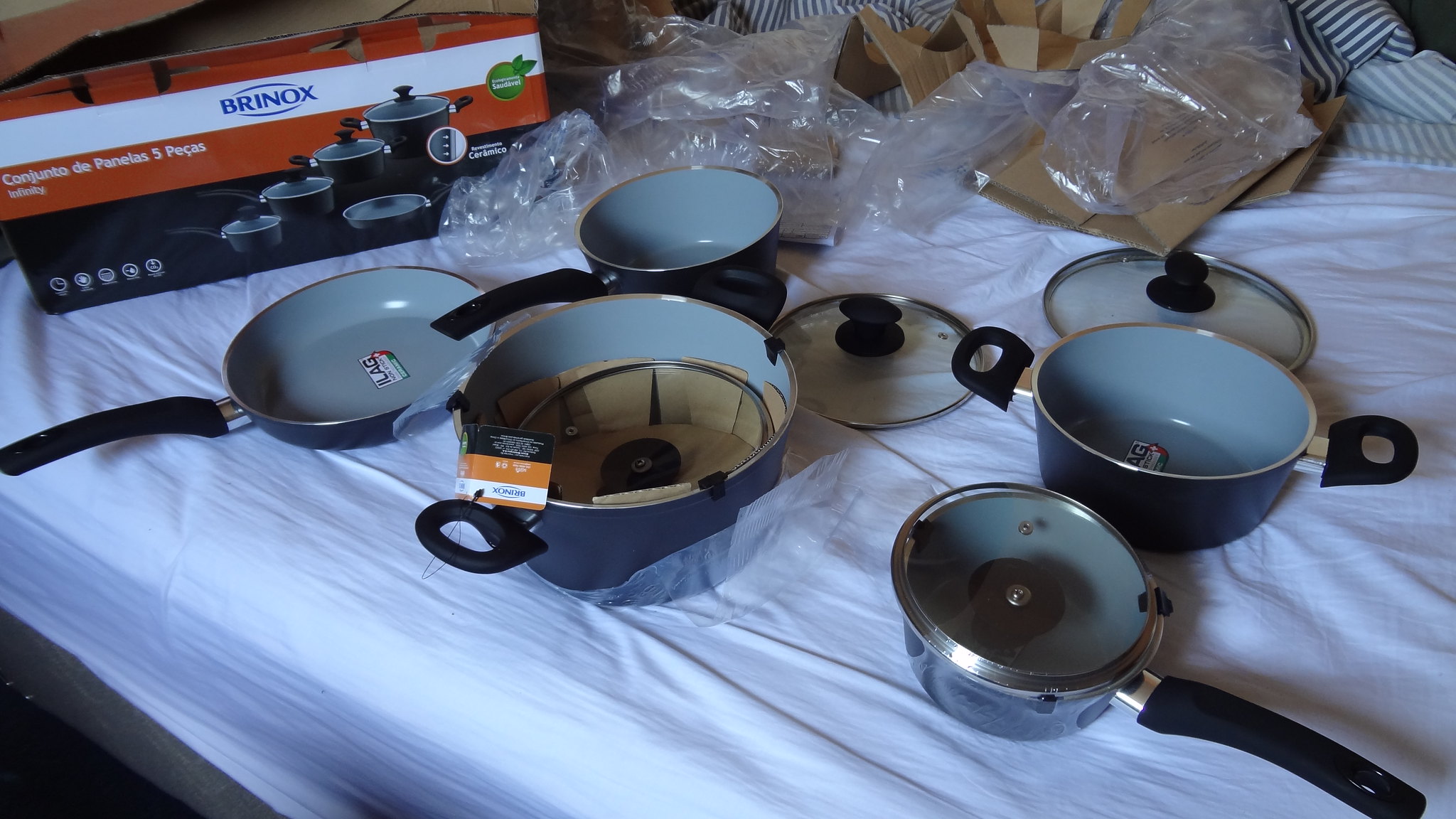The image depicts an unboxing scene of a brand new Brinox pan set, spread out on a table covered with a white sheet. The set includes five pieces: a large Dutch oven, a frying pan, and three different-sized pots, all in a coordinated design with dark blue exteriors, light blue interiors, and black handles. Each pot comes with a glass lid featuring a black knob, except for the frying pan which has no lid. In the upper part of the image, the red, white, and black packaging box is visible, displaying images of the cookware and the brand name, Brinox, prominently written in blue font. Scattered around the tabletop are various packing materials, including plastic wrap and cardboard, indicating that the items have just been unpacked. There is also some confusion about the setting, suggesting it might actually be a bed with a white sheet rather than a table.